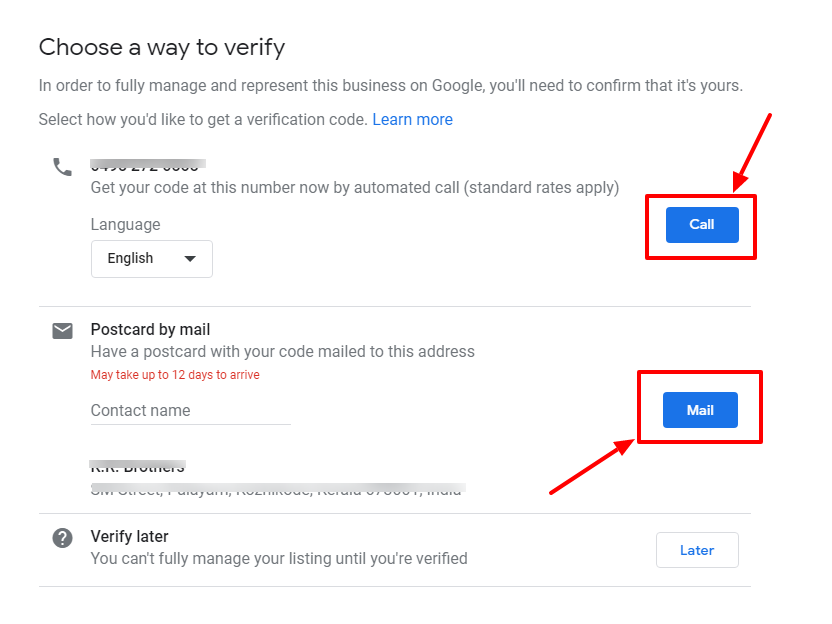This instructional image is a screenshot from a website detailing how to verify ownership of a business on Google. At the top left, the title "Choose a Way to Verify" is prominently displayed in black text. Directly below, in gray text, it states, "In order to fully manage and represent this business on Google, you will need to confirm that it's yours. Select how you'd like to get a verification code," followed by a blue, hyperlinked "Learn more."

The image visualizes multiple verification options:

1. **Phone Verification**:
    - A phone icon is presented alongside a grayed-out placeholder for a phone number to ensure privacy.
    - Instructions read, "Get your code at this number now by automated call (standard rates apply)."
    - A blue, clickable "Call" button is circled in a red rectangle with a red arrow pointing to it, drawing attention to this option.
  
2. **Language Selection**:
    - On the left, there's a dropdown menu labeled "Language" with "English" selected as the default. This indicates that the user can choose other language options if needed.

3. **Postcard by Mail Verification**:
    - Instructions read, "Have a postcard with your code mailed to this address, may take up to 12 days to arrive."
    - Another red box around a blue "Mail" button is highlighted with a red arrow, emphasizing this option.
    - Additional information under this section has been grayed out to maintain privacy.

4. **Verification Later**:
    - Marked by a question mark in a circle.
    - The text indicates, "You can't fully manage your listing until you've verified," with a smaller clickable "Later" button in blue.

The two primary verification options—phone and mail—feature notable blue buttons with white text, emphasizing their readiness for user interaction.